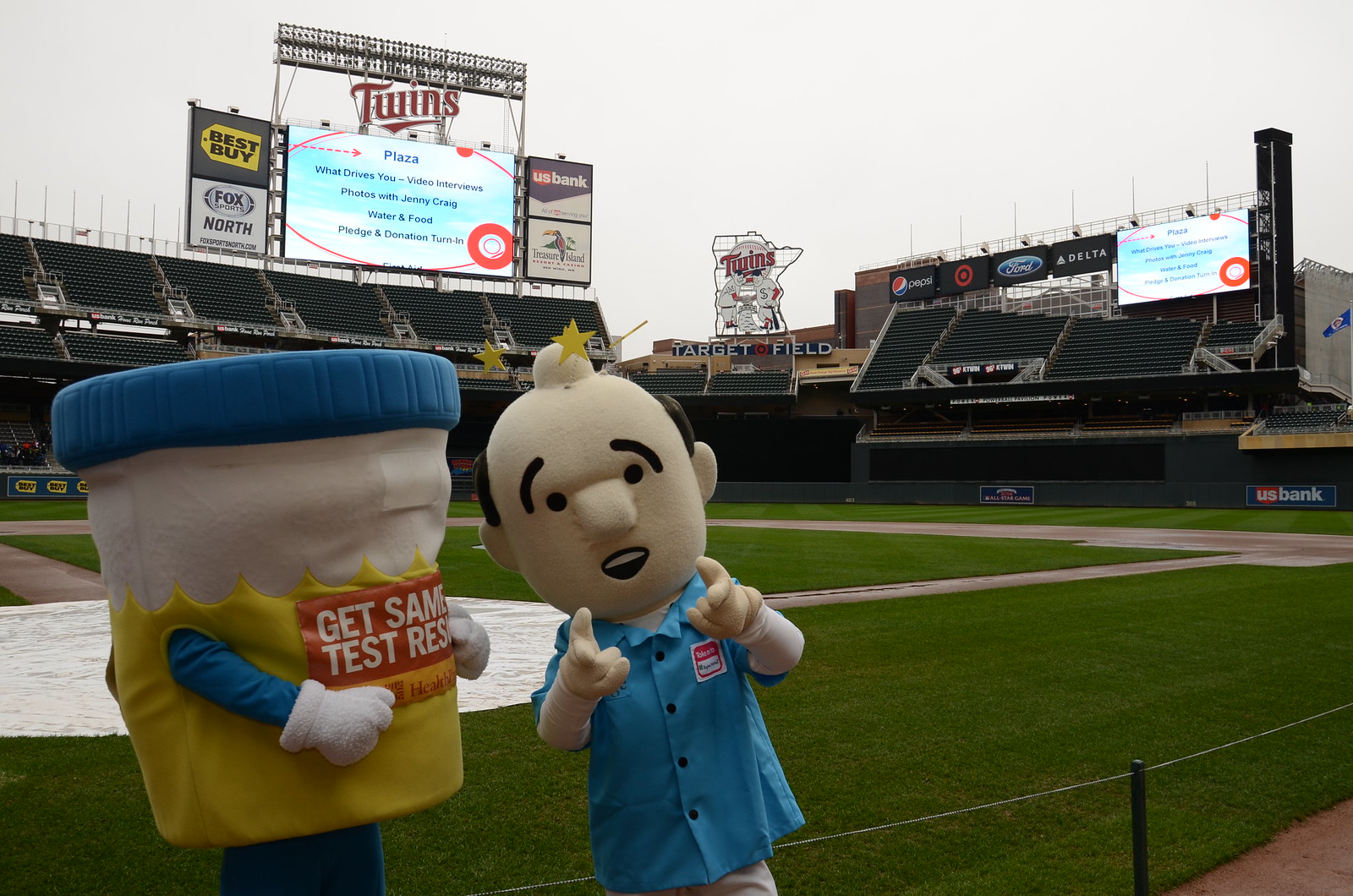The image showcases Target Field, home of the Minnesota Twins, on a cloudy day. The scene is devoid of fans, with the green field and empty bleachers creating a tranquil atmosphere. Prominent advertising banners are displayed around the stadium, including US Bank, Best Buy, Fox Sports, Ford, Delta, Pepsi, and Treasure Island. A large monitor in the background displays "Twins Plaza," alongside messages like "What Drives You," "Video Interviews," and "Photos with Jamie Greig," surrounded by additional branding. Two mascots are the focal point of the image: one is a man in a blue shirt, balding, pointing at the camera, possibly representing a pharmacist, while the other mascot resembles a collection jar with a blue top, white and yellow body, blue pants, and white gloves, bearing the red text "Get Same Test Results."